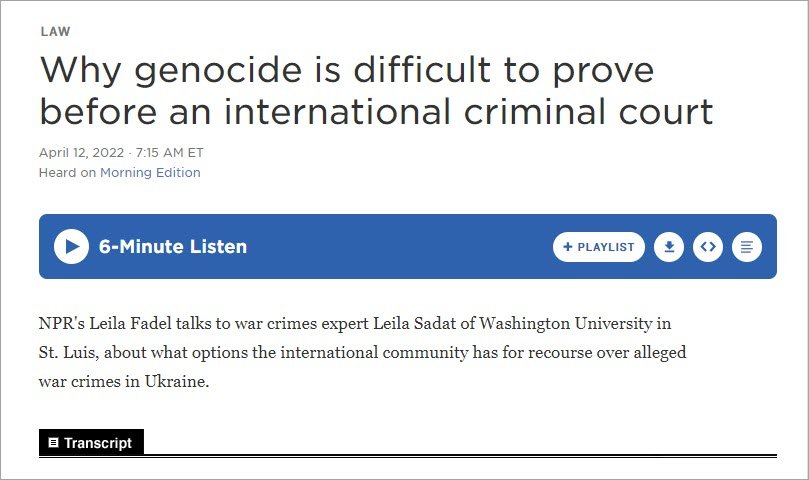This image depicts a screenshot from a website that hosts audio clips. The layout is characterized by a thin black border surrounding the main content against a white background. In the top left corner, the text reads "law law.law."

Prominently displayed is the title, "Why Genocide is Difficult to Prove Before an International Criminal Court," with a publication date of April 12th, 2022, at 7:15 a.m. Eastern Time. The source of this content is "Morning Edition."

Below the title, a blue bar features a white play button on the left side, indicating that it is a "six-minute listen." On the right side of the blue bar, a white speech bubble icon marked "Playlist" allows users to add the content to their playlist. Additional icons for download, embed, and a list-like paper icon are also present, facilitating various interactive options.

Beneath this bar, there is a brief introduction about Leila Fidel, outlining the main topics discussed in the audio clip.